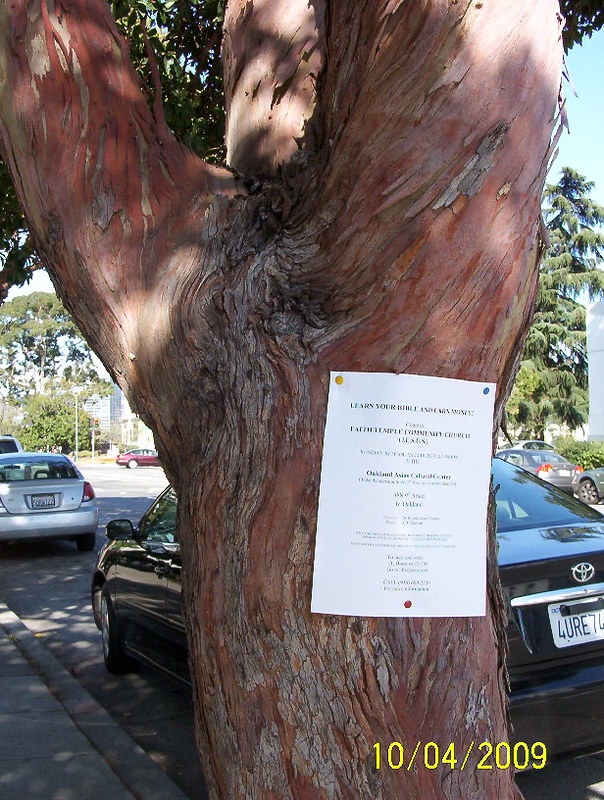The image, taken on October 4th, 2009, showcases a large tree with a broad trunk and three main branches, centrally positioned on a city sidewalk. The tree's bark appears somewhat scratched up, and a notice is pinned to it, although the text on the paper is unreadable due to the photo's low resolution. The notice seems to be a white sheet with black printed text, held in place by yellow, blue, and red thumbtacks. In the background, the scene extends to a sunny, cloudless day featuring a city street lined with parked cars, including a black Toyota with a California license plate directly behind the tree and other cars like a silver one on the left and a maroon one further back. Several buildings and additional trees are visible further down the street, completing the urban backdrop. The bottom right of the photograph bears a yellow watermark indicating the date "10/04/2009."